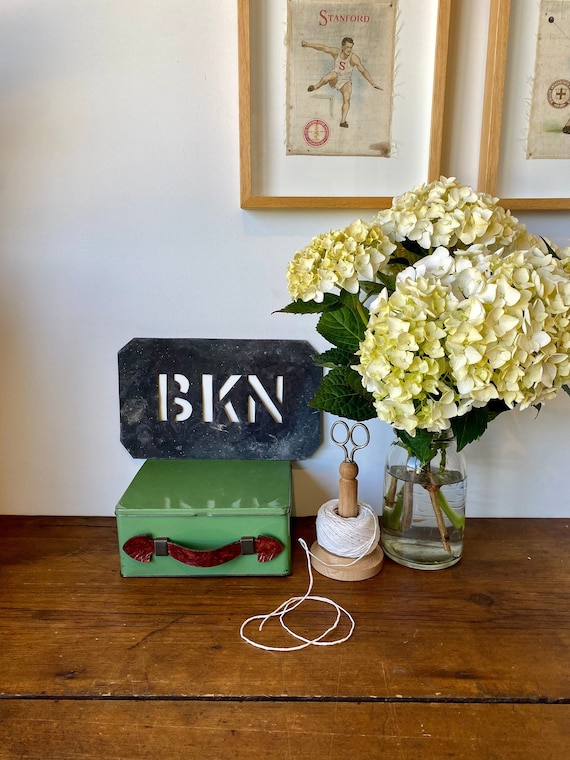This color photo showcases a wooden surface, possibly a table or counter, and a variety of items arranged against a white wall. On the wall, there are two framed images that are partially visible. One clearly depicts an athlete, a man mid-jump, with the word "Stanford" printed prominently. The frames are taller than they are wide, suggesting a portrait orientation.

On the surface below, several items are carefully arranged. To the right sits a clear jar vase holding a lush bouquet of yellow flowers, likely hydrangeas, known for their large, poofy clusters that resemble popcorn. Adjoining it is a spool of white yarn, with a pair of scissors inserted into it, indicating its use. Next to these items is a green suitcase or chest, adding a touch of vintage charm to the scene. Finally, there is a black and white sign with the letters "BKN," placed on or near a gray metal box, which some might speculate is a cash box.